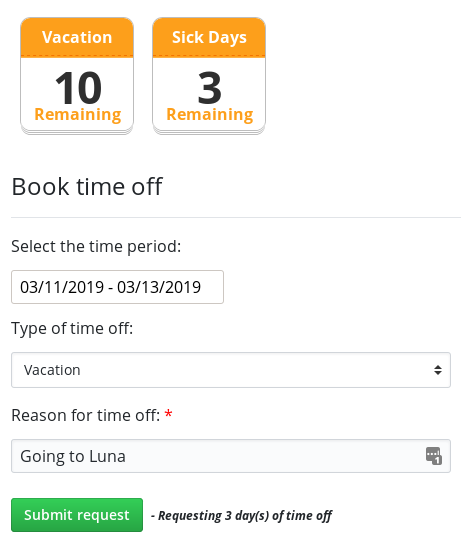The image depicts an online form designed for requesting days off from work. The background is white, providing a clean interface. At the top, there are two calendar-style icons. The first icon has a yellow header that reads "VACATION" in white text. Beneath this header, a white box displays the number "10" in black, indicating the number of vacation days available. Below the white box, the word "REMAINING" is written in yellow.

The second calendar icon follows a similar format. Its yellow header reads "SICK DAYS" in white text. The white box below this header shows the number "3" in black, with the word "REMAINING" in yellow underneath.

Below these icons, a larger section of the form titled "Book Time Off" is written in black text. This title is underlined with a thin gray line. Beneath this, smaller black text instructs users to "Select the time period:" followed by a rectangular box where the user can input dates. In this instance, the dates range from "03/11/2019" to "03/13/2019."

Directly under the date selection box, another section labeled "Type of Time Off:" is located. A drop-down menu box displays "Vacation" as the selected type of time off. To the right of this box are up and down arrows for scrolling, both in black.

Further down, another label reads "Reason for Time Off:" accompanied by a red asterisk, indicating that this field is required. Below this, a text box contains the words "Going to Luna." An icon resembling a calendar with a white number "1" pops out from the right side of this text box.

At the bottom of the form, a green rectangular button labeled "Submit Request" in white text is positioned to the left. To its right, smaller black text notes "- requesting 3 days of time off," with the 's' in parentheses.

Overall, the form is structured for users to efficiently request time off, with clear sections and easily identifiable input fields.